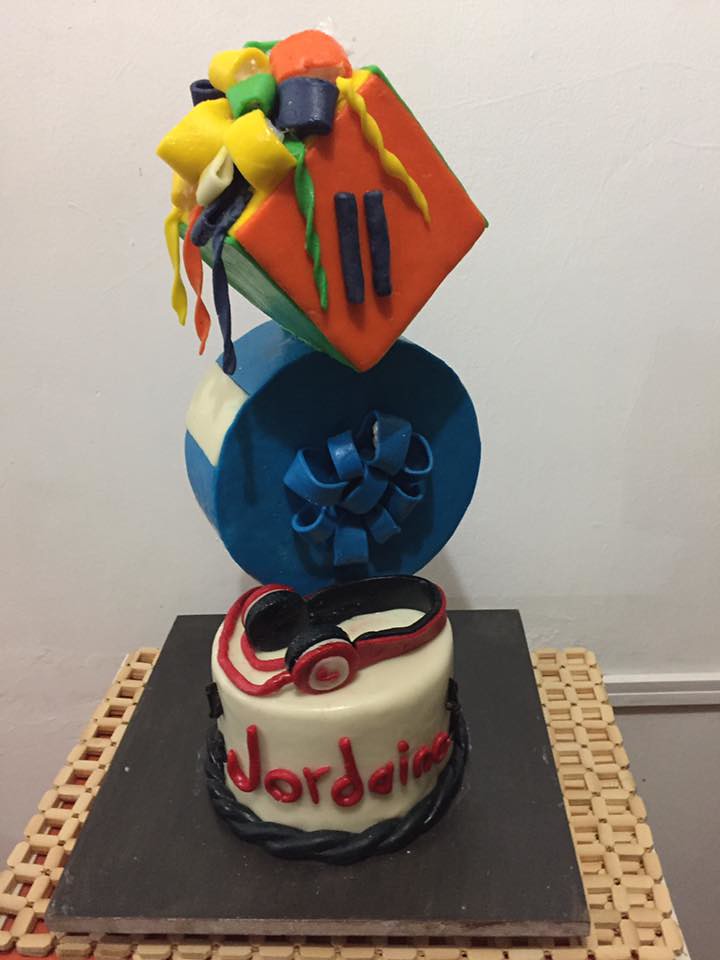The image showcases a creatively designed, three-tiered cake placed on a black square platform atop a wooden table. The table's surface appears to be an intricate mosaic of small, glued-together squares, with hints of orange peeking through. The cake has a white base layer with "Jordan" written in red icing, encircled by a twisted black rope-like decoration. The second tier is a blue fondant circle adorned with a white stripe and a bow, giving it the appearance of a wrapped present. Crowning the cake is an orange and green present-shaped tier that lies on its side, embellished with colorful ribbons and streamers in shades of yellow, green, purple, and orange, along with two purple lines. Red and black headphones made of fondant rest on the top layer, adding a playful touch. The background features a plain white wall and a gray floor, directing attention to the elaborate cake and its unique design elements.